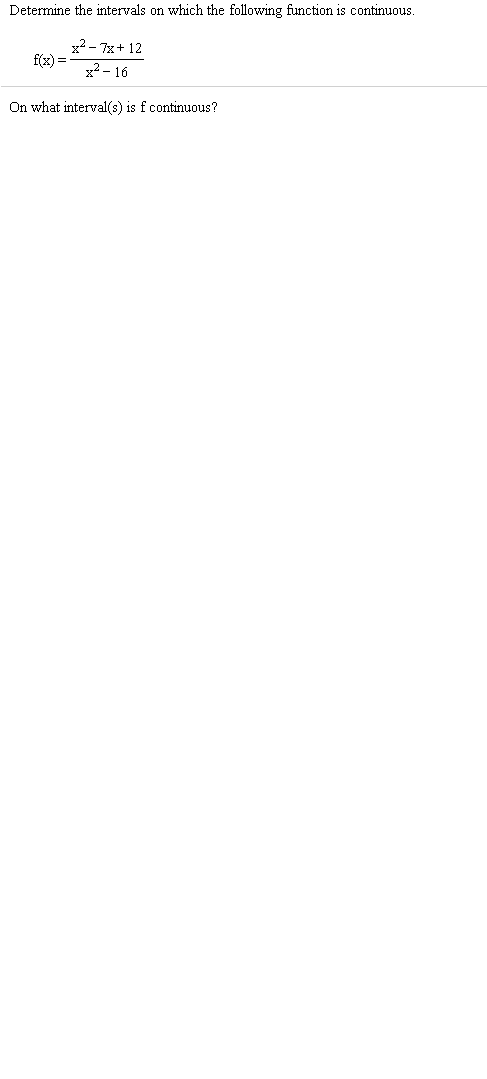A mathematical formula is presented on a white background. The equation is straightforward, appearing as though it might have been typed on a piece of paper or extracted from a web page. Despite the relatively small print, the text remains legible. The task is to determine the intervals on which the given function is continuous. 

The function is defined as \( f(x) = \frac{x^2 - 7x + 12}{x^2 - 16} \). Below the function, there is a delicate line followed by the instruction: "On what interval(s) is \( f \) continuous?"

The equation falls under algebra, featuring a quadratic numerator \( x^2 - 7x + 12 \) and a quadratic denominator \( x^2 - 16 \). The formula comprises various mathematical elements, including variables, exponents, and arithmetic operations like addition and subtraction.

Overall, the presentation of this equation is reminiscent of traditional typesetting rather than modern computer fonts, given its simple black text on a white background. This algebraic expression serves as a reminder of the kinds of problems often encountered during school mathematics lessons, albeit not frequently applied in everyday tasks such as balancing a checkbook.